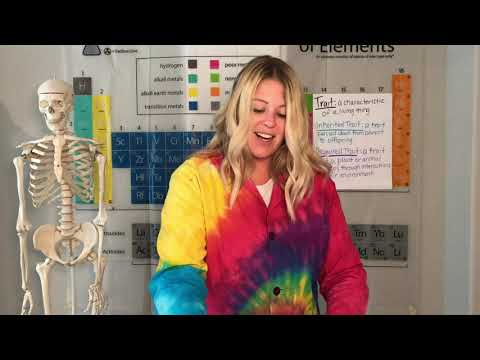The image captures a science classroom scene centered on a woman who seems to be either a student or a teacher, likely in a chemistry or biology setting. She is a young Caucasian, with bleached blonde hair accented by dark roots, her hair extending just past her shoulders, slightly curled at the ends. She has a pleasant expression, smiling or talking while looking straight down. She is attired in a vibrant tie-dyed button-down smock, displaying an array of colors including blue, yellow, red, purple, and green, over a white shirt. Behind her, the background features a large multicolored periodic table poster with blue and white writing. Additionally, a skeleton is visible hanging from a rack to her left. The edges of the photograph have plain black headers and footers, providing a clear frame for the scene.